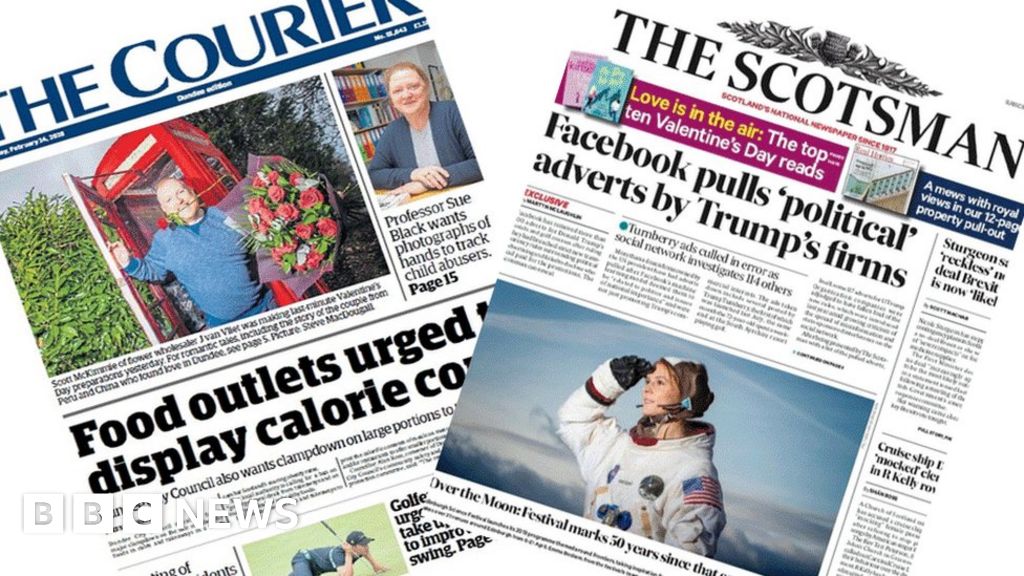The image depicts a variety of newspaper front pages with detailed headlines and images. One prominent newspaper features “The Courier” in navy blue font with white text. It includes a photograph of a portly gentleman inside a red phone booth, holding a bouquet of reddish flowers and a rose clenched between his teeth. The man is dressed in a blue shirt. The headline, though slightly blurry in black font, mentions “Scott McKinney.”

Adjacent to this is another notable headline: “Professor Sue Black wants photographs of hands to track child abusers on page 15.” This headline is accompanied by an image of a stern-faced woman with her hands on a table, dressed in blue.

Another newspaper displayed is “The Scotsman,” which claims to be “Scotland's national newspaper” since a specific year printed in red. One banner on this paper reads, “Love is in the Air: The Top 10 Valentine's Day Reads,” featuring book covers in yellow, teal, pink, and white. Another banner states, “A Muse with Royal Views and Our 12-Page Property Pullout.” 

A notable black headline on this paper reads, “Facebook Pulls Political Adverts by Trump Firms: Turnberry Ads Cold and Air Social Network Investigates 114 Others,” followed by several paragraphs of text. There are also various other headlines and an image of a female astronaut dressed in uniform. The intricate composition captures the diversity and depth of current events and features presented across multiple newspapers.